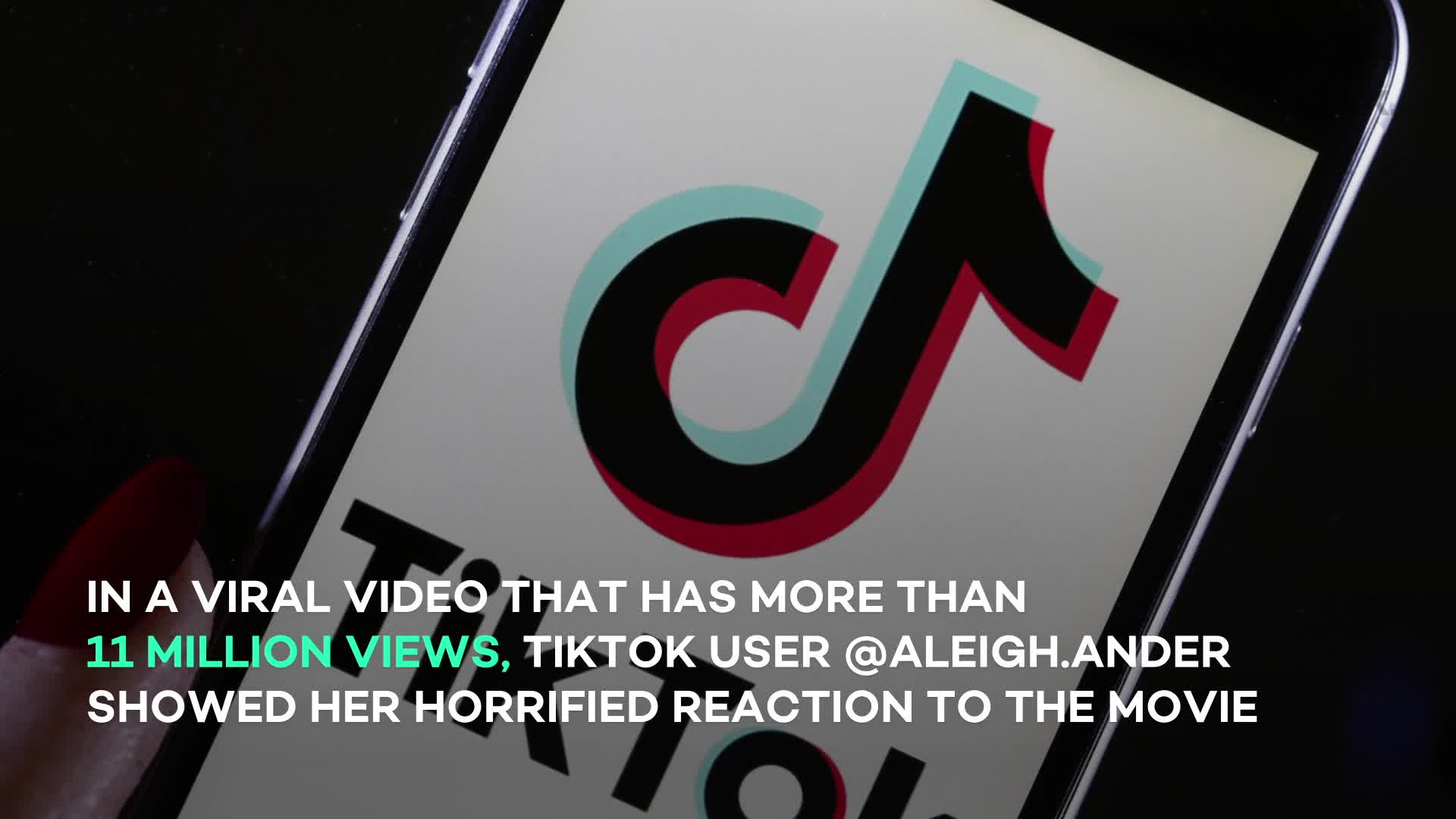In the image, a left hand holds a smartphone at a 45-degree angle from southwest to northeast, completely filling the screen with the TikTok symbol. The symbol is depicted in a layered fashion with a backdrop of teal/mint green and a superimposed red, creating a visually striking effect where parts appear black due to the offset alignment of the colors. Below the symbol, the text "TikTok" is clearly visible. Superimposed across the image in white text, a message reads: "In a viral video that has more than 11 MILLION VIEWS, TikTok user @ali.and.er showed her horrified reaction to the movie." The view count "11 MILLION VIEWS" is highlighted in mint green, emphasizing its significance.